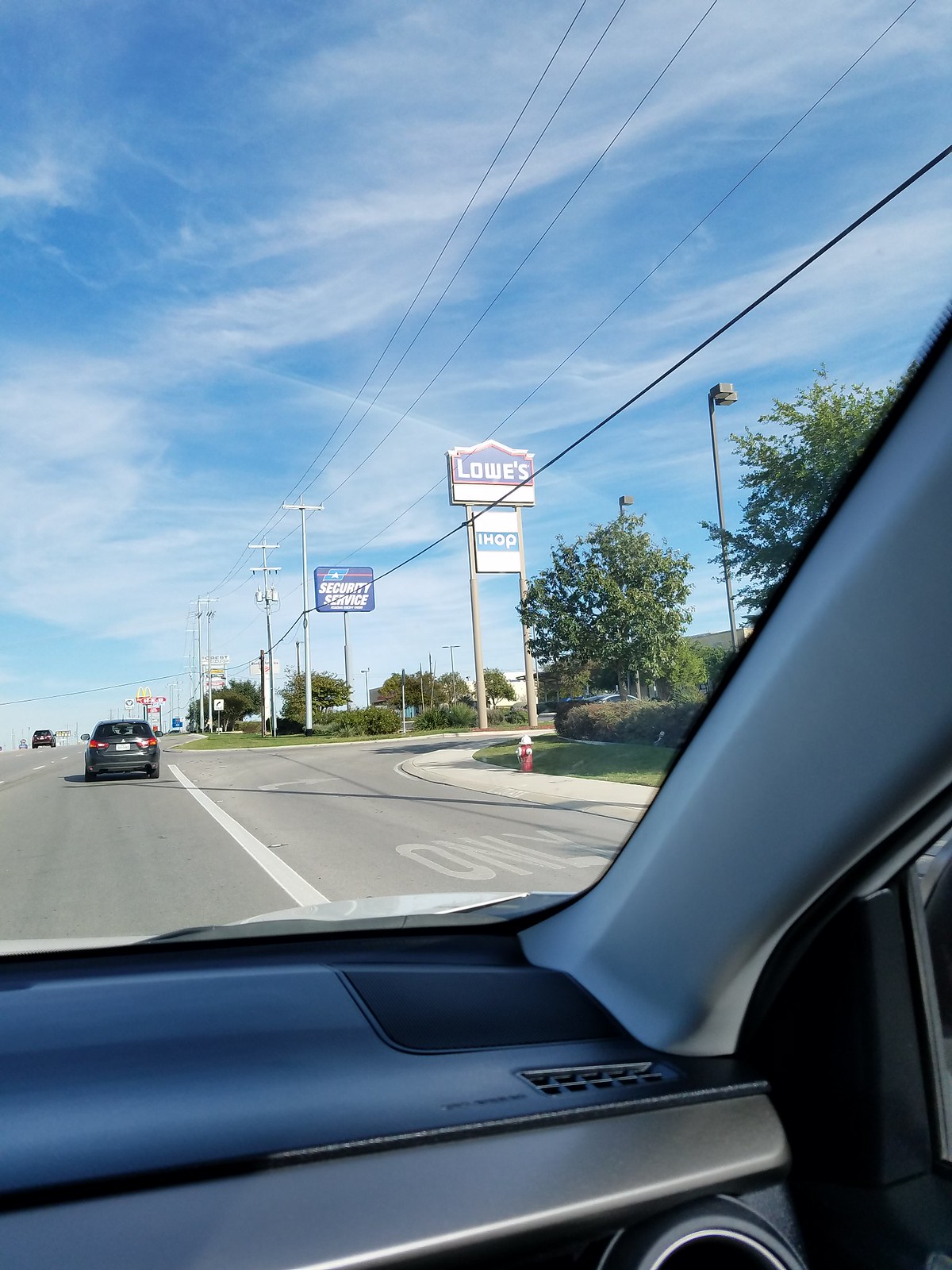This image, taken from the interior of a car on a light gray asphalt road, captures a bustling shopping area under a blue sky with white clouds. The photo, shot from the passenger side perspective, reveals part of the car's interior with a black dashboard and a light gray pillar. Stretching ahead is a road marked with a white arrow pointing right and the word "ONLY," indicating a right turn only lane.

Prominently, there are several signs that indicate businesses in the vicinity: a large blue sign for Lowe's, a white sign with a blue banner for IHOP, and another blue sign further back reading "Security Service." In the distance, the golden arches of McDonald's are visible. Power lines crisscross the scene, and traffic is evident with several cars on the road. To the right, there are additional features such as streetlights, a sidewalk, a red fire hydrant with a white cap, and some green hedges, enhancing the detailed urban setting captured by the dashcam.